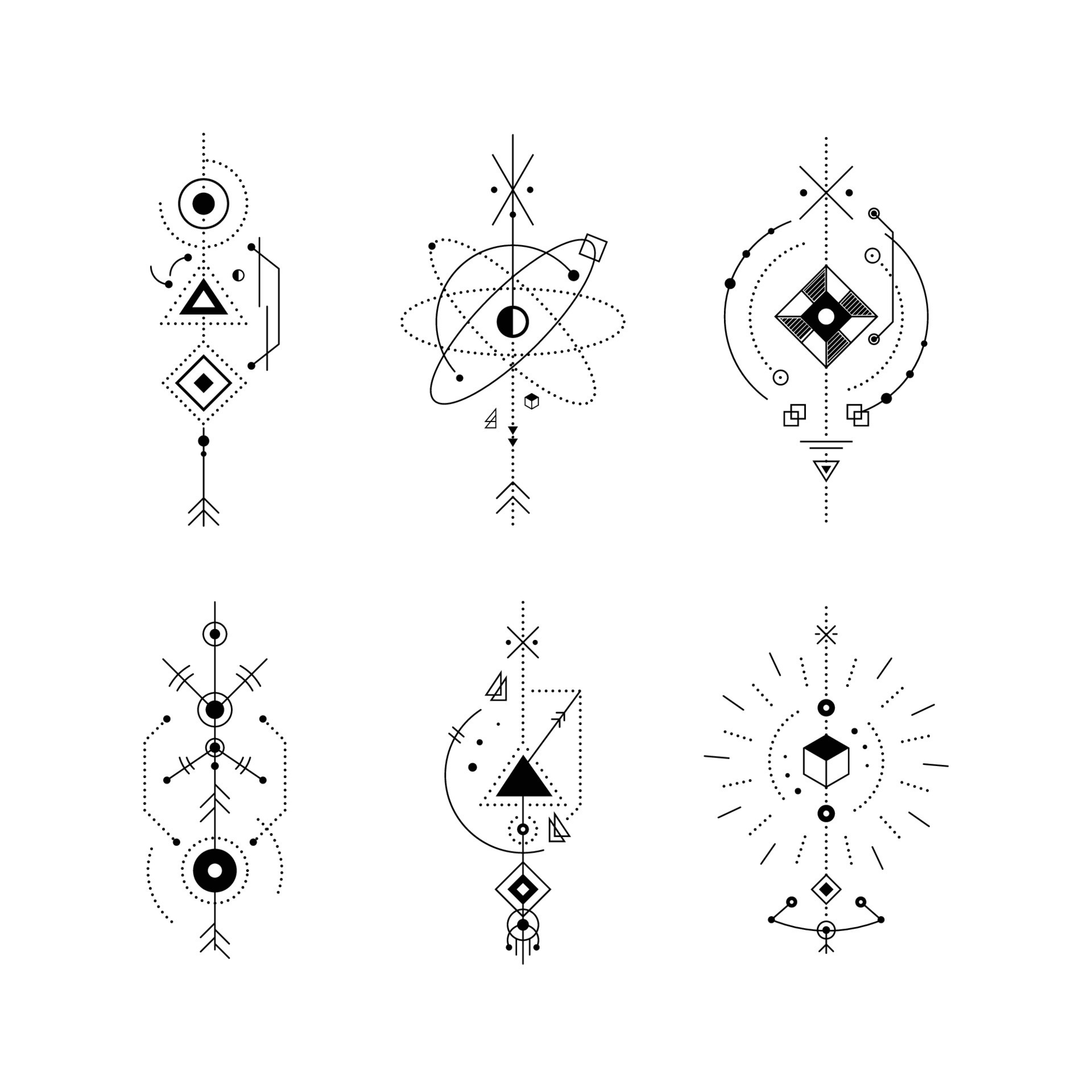This image features six distinct black geometric designs against a white background, meticulously crafted to resemble potential tattoo art. Arranged in two rows of three, the designs feature an array of shapes including circles, triangles, squares, and arrows. The top row starts with a pattern comprising triangles, squares, circles, and arrows. The central design in this row incorporates ovals, circles, and lines, followed by a design featuring squares, circles, and lines. In the bottom row, the first design includes lines at 45-degree angles, circles, and arrows. The next design displays a mix of triangles, squares, circles, and lines. The final design on the bottom row showcases a cube, triangles, circles, and lines. The intricate compositions include elements resembling atoms with electrons in orbit, alongside dotted lines and curves, creating a complex and ornate appearance suitable for tattoo motifs.